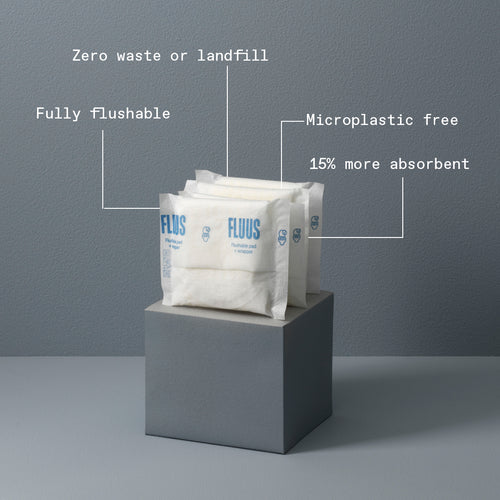The image depicts a minimalist scene with a gray cube situated on a matching gray surface, set against a textured, gray-painted wall. Atop the cube are four rectangular white packets that display the brand name "FLUUS" in blue letters. These packets are prominently highlighted by various labels in white text that are connected by lines. The labels describe the product features, stating "Zero waste or landfill," "Fully flushable," "Microplastic free," and "15% more absorbent." The lighting in the image is bright, accentuating the clarity and details of the scene.